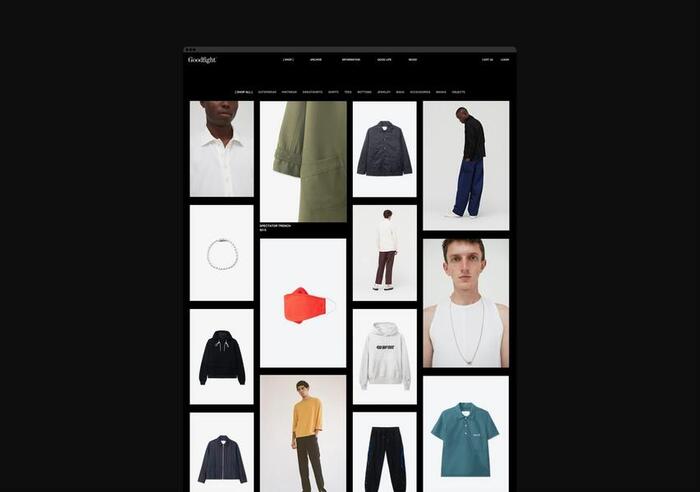The image showcases a website page designed for a menswear retailer called "Young Men." The layout features a sleek black background with a top navigation bar in small print, offering various clickable categories. The centerpiece of the page is a collection of diverse clothing items and models, each contributing to a meticulously curated fashion ensemble.

Prominent images include:
- A pristine white, button-up shirt with a collar, neatly buttoned up except for the top button.
- A glimpse of a green coat or jacket, revealing just the back and one sleeve.
- A classic blue denim jacket.
- A young man dressed in blue pants paired with a black top.
- Another model with his back to the viewer, wearing brown pants, a white top, white shoes, and sporting black hair along with a silver bracelet.
- Two jackets located in the lower left, one black and the other blue.
- A young man clad in a yellow sweatshirt and brown pants.
- A solitary pair of black pants and a separate blue-green short-sleeve polo shirt.
- A white sweatshirt adorned with black print across the front.

Additionally, there is a young man featured in a white sleeveless t-shirt, accessorized with a silver necklace. He has short black hair, further adding to the stylish diversity of the collection displayed on this menswear site.